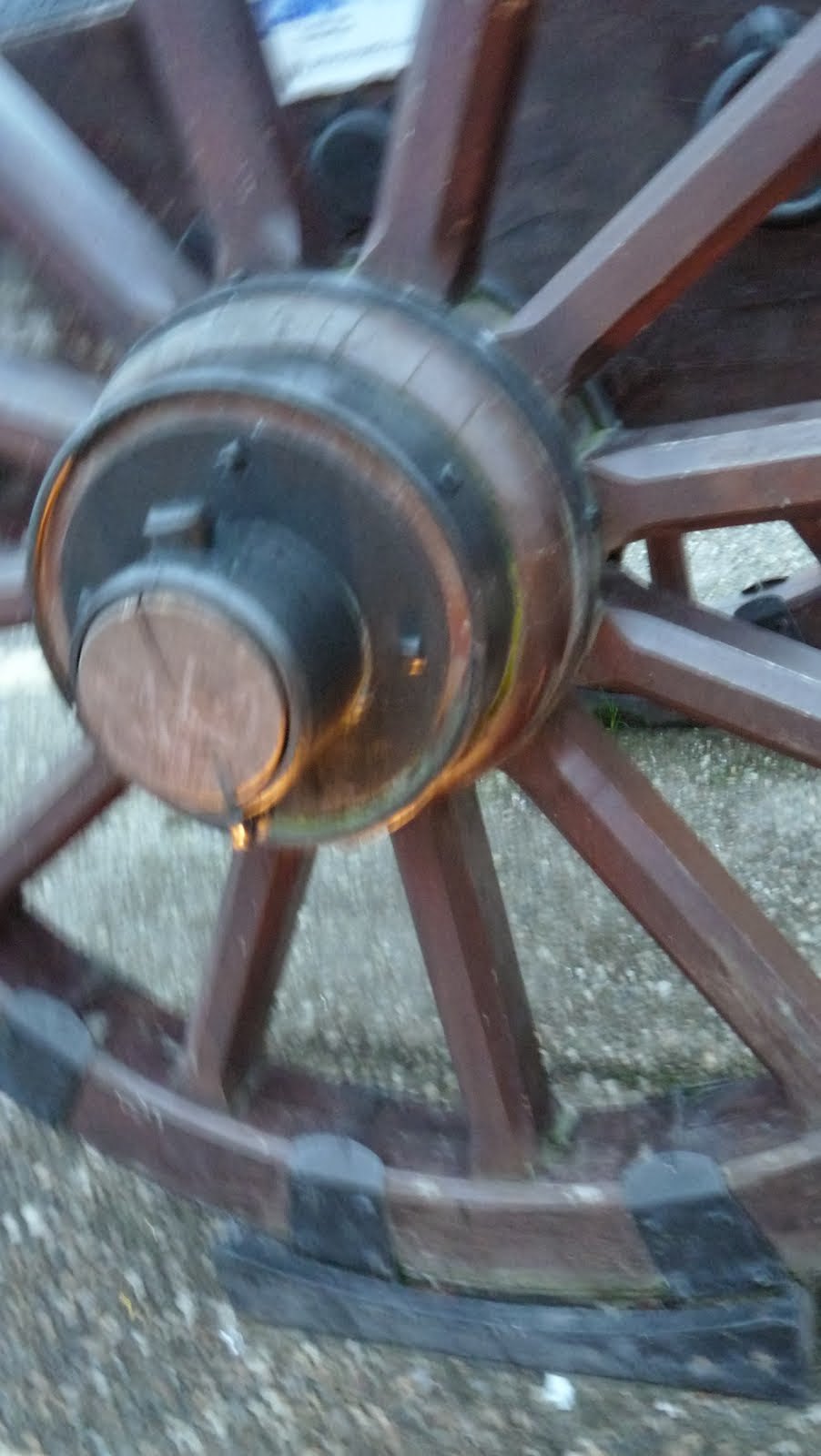This image captures a close-up of an old-fashioned wagon wheel, displaying a stationary state. The wheel is primarily wooden with a light brown barrel at its center, from which twelve to thirteen darker brown wooden spokes radiate outward. Each spoke transitions seamlessly into the same dark brown hue that continues around the wheel's rim. Metal casings are interspersed between the spokes, providing structural reinforcement. The hub is encased in metal bands, adding to the aged and rustic appearance of the wheel. The entire assembly is pinned in place by a metal post protruding from the ground, likely part of a permanent display. This entire scene is set against a gravel ground composed of various pebbles, contributing to the wheel's antique charm. The image is quite blurry and muted, giving it a nostalgic and subdued atmosphere.